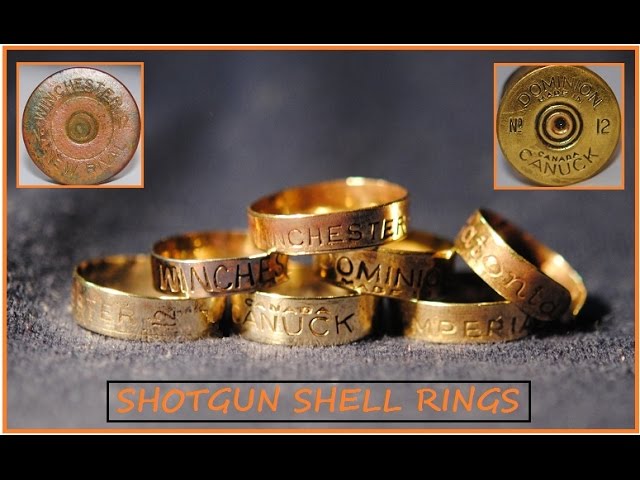The image depicts a promotional photo of seven golden shotgun shell rings arranged centrally on a gray fabric background. These rings, resembling wedding bands with a thicker diameter, have various inscriptions such as "Winchester," "Canada Canuck," "Dominion," and possibly "Imperial." The golden rings are meticulously placed one on top of another, displaying their engraved details. The photograph is framed with a thin orange border and features an inset on the top left and right corners displaying close-ups of two different shotgun shell casings. The left casing, slightly weathered, clearly reads "Winchester," and the right, newer casing, states "Canada Canuck" and "Dominion 12." At the bottom of the photo, within a black box with orange text, the words "shotgun shell rings" are prominently displayed. The image's backdrop is a solid black, creating a stark contrast to highlight the intricate details and luster of the golden rings.